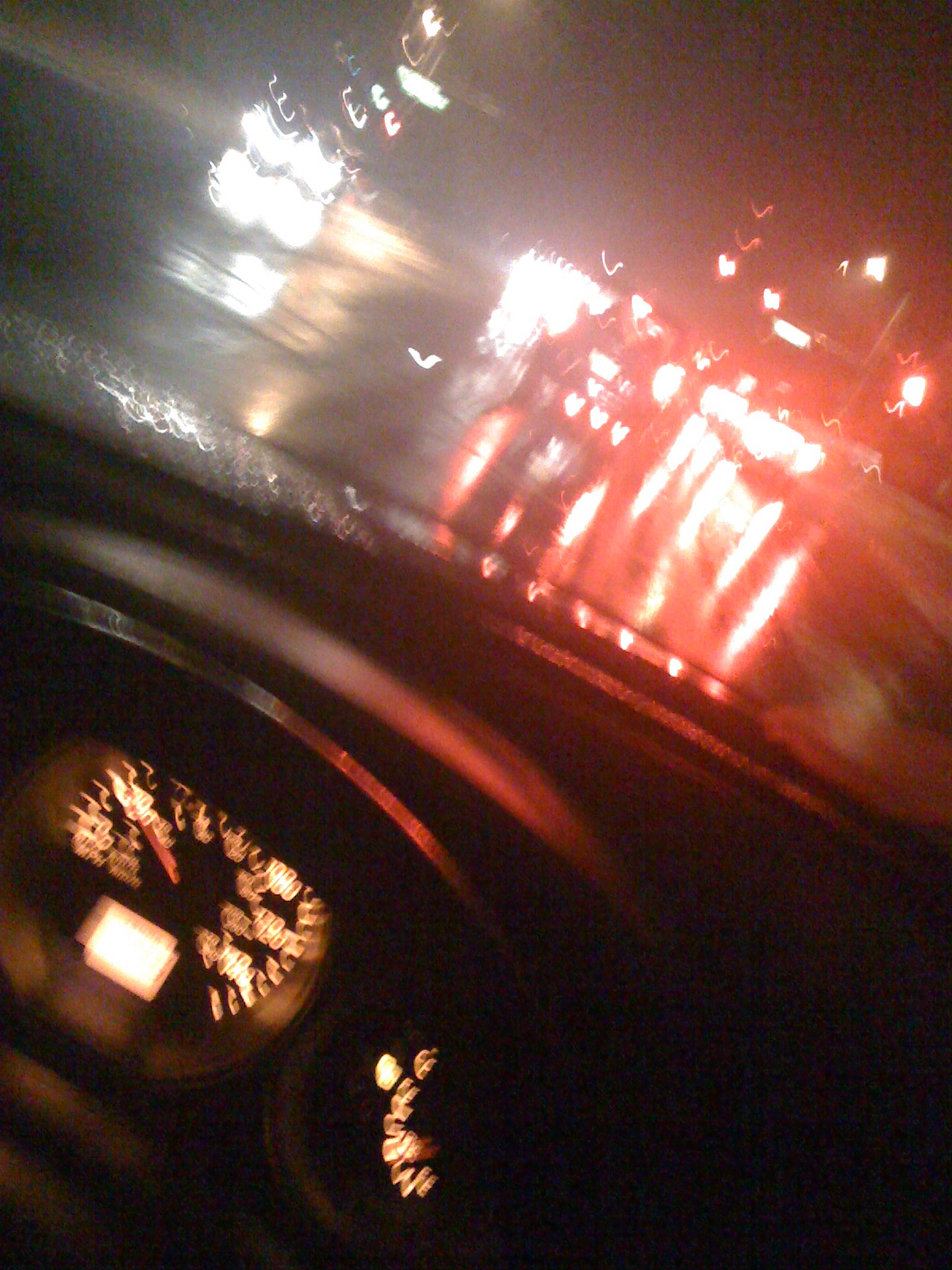From the perspective of the driver's seat, this blurry and out-of-focus photo captures a rainy intersection at night. The top of the steering wheel is visible, along with the illuminated speedometer and another gauge to its right. Raindrops distort the view through the windshield, turning the lights of the cars ahead into indistinct blurs. The traffic signal ahead shines red for the lanes to the right, while oncoming traffic is visible in the opposite lanes. The darkness of night envelops the scene, and the angle of the shot gives the impression that the car is slightly askew.